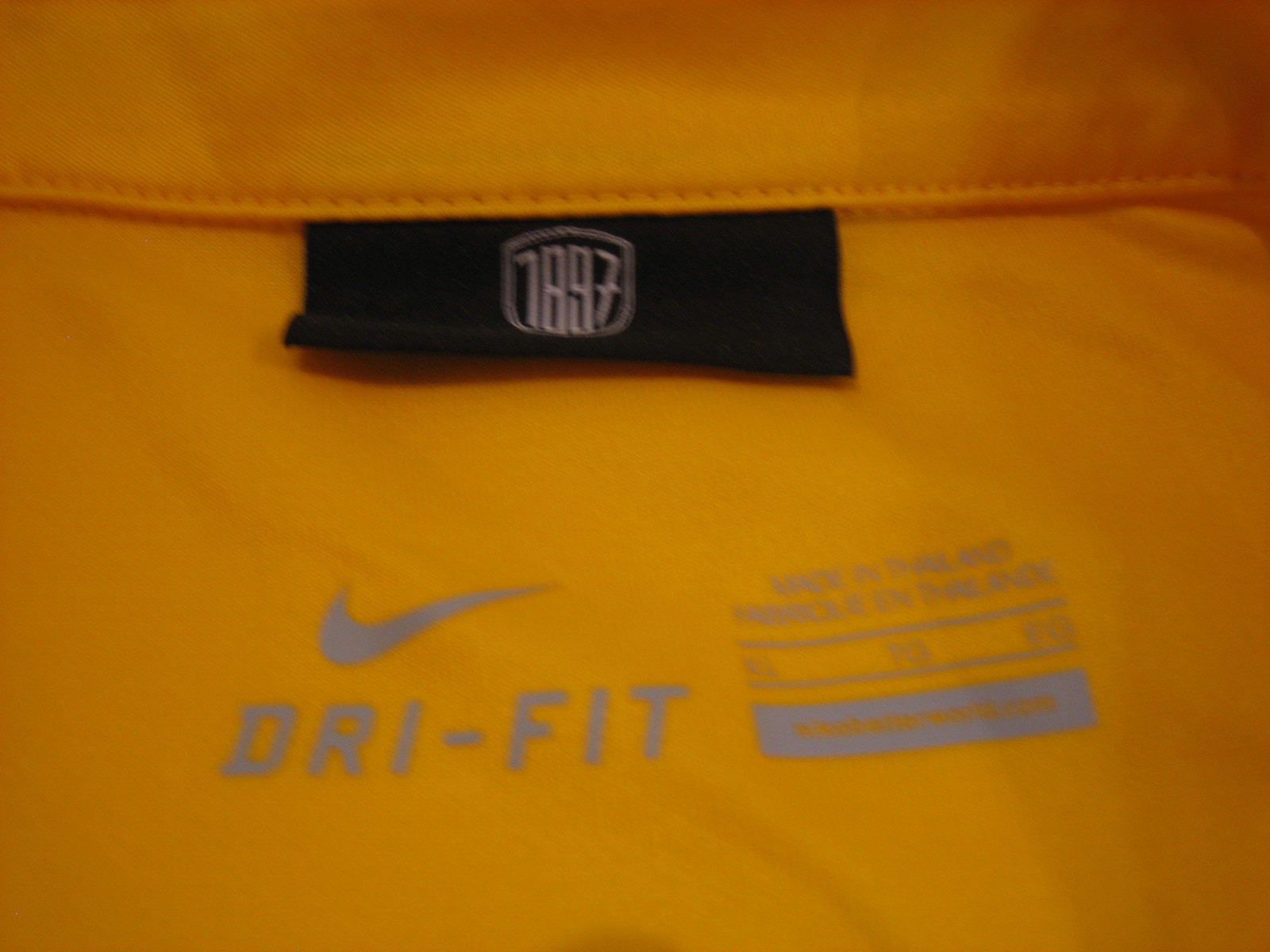This image provides a detailed close-up view of the inside of a bright orange Nike sports shirt, focusing on the area around the neck and upper chest or back. The shirt features a black rectangular tag in the center, from about two inches to the left to two inches from the right, with white stitching displaying the numbers "1897" prominently in the middle. Below the tag is printed the Nike logo and "DRI-FIT" in capital letters, displayed in a grey-silver color. Adjacent to the "DRI-FIT" text, it states "Made in Thailand" and its French translation "Fabriqué en Thaïlande," also in grey lettering. Additionally, there's a small, blurry section that appears to provide size information, which may indicate the shirt is a large (L). The label area includes stitching in black and an orange round border, blending into the shirt's overall bright orange fabric.